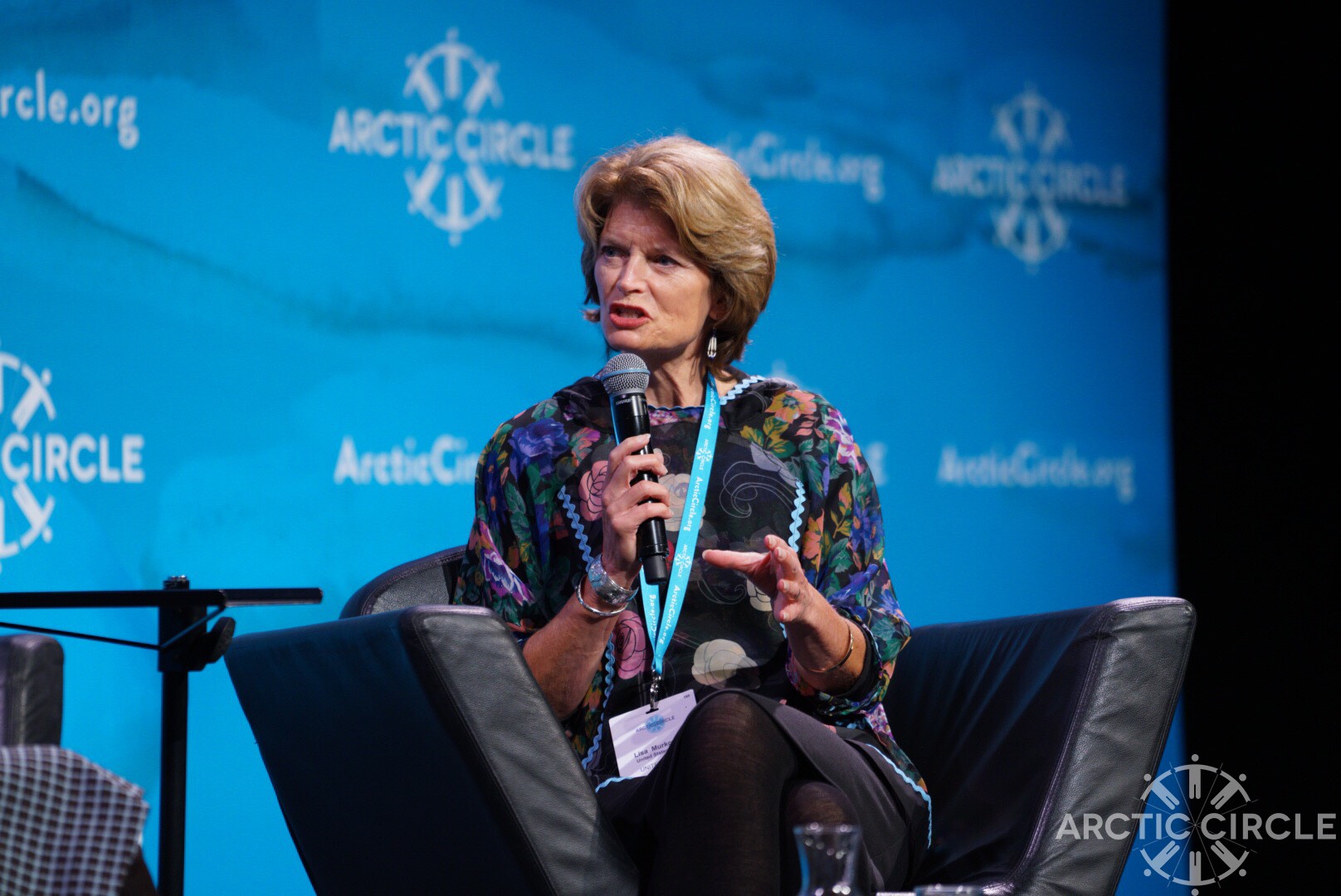The image features Alaska Senator Lisa Murkowski speaking at a conference. She is seated in a black leather chair on stage, addressing the audience with a wireless microphone held in her right hand, her mouth open as she speaks. Senator Murkowski is wearing a colorful floral top paired with black slacks, accessorized with a light blue lanyard and a white name tag around her neck. She also wears bracelets and has medium-length, fluffy blonde hair with visible brown undertones at the back. Her serious expression suggests she is engaged deeply in her speech. Behind her, a large screen and the stage backdrop both prominently display the Arctic Circle emblem, which consists of six silhouetted figures arranged in a circle around the text "Arctic Circle" set against a blue, icy background. Additionally, a water glass and a dispenser are visible on a table in front of her. The lower right corner of the image features a watermark of the Arctic Circle emblem.